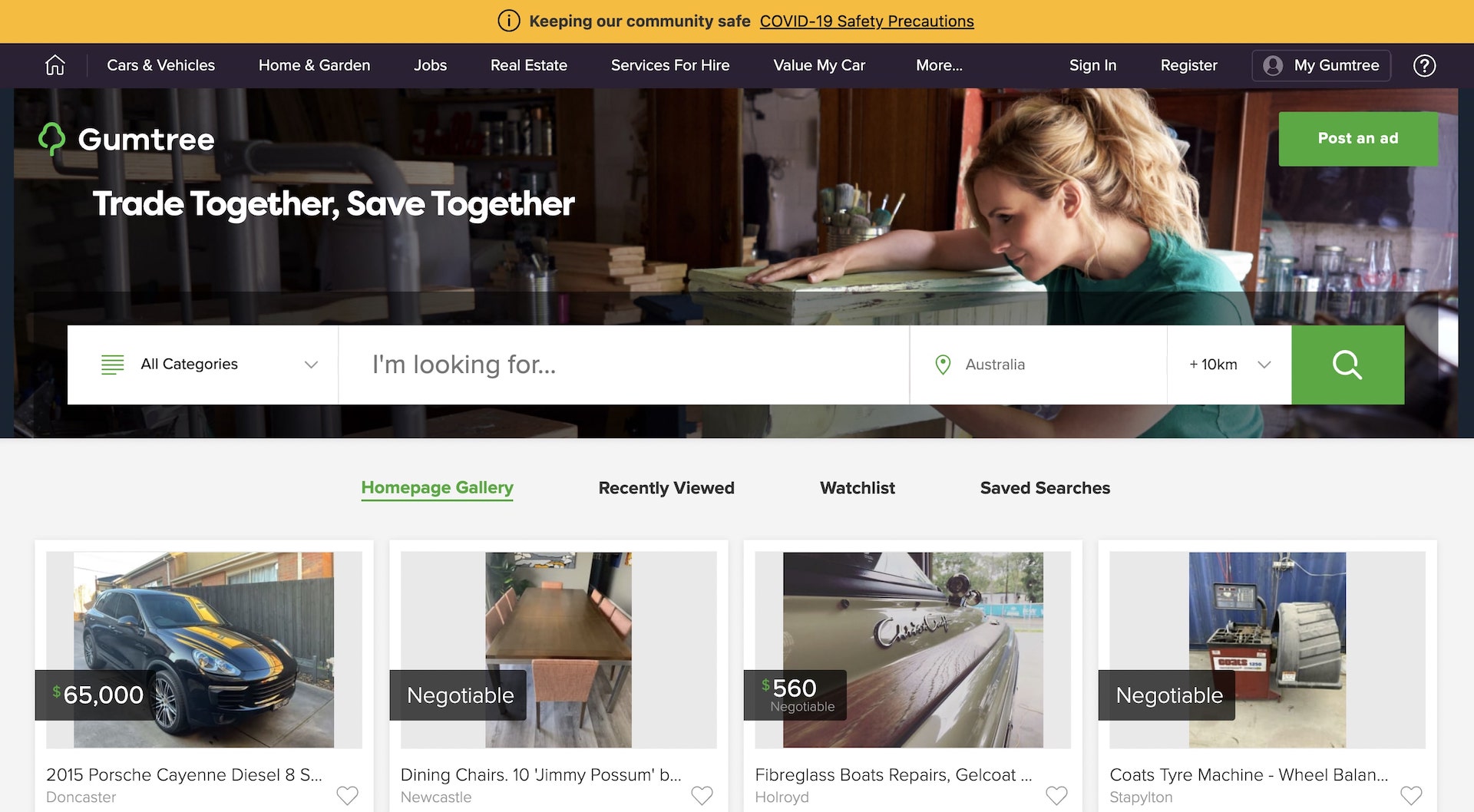The homepage of the Gumtree website is designed to facilitate the buying and selling of a wide array of items. At the top of the webpage, a generic image features a young blonde woman with a pigtail, wearing a green shirt, who is either contemplating a potential purchase or admiring a recent acquisition. The site’s name, Gumtree, is prominently displayed in the top left corner along with the tagline "Trade Together, Save Together."

The navigation bar spans the top of the page, offering various categories including "Cars & Vehicles," "Home & Garden," "Jobs," "Real Estate," "Services for Hire," "Value My Car," and a "More" option for additional, less commonly accessed categories. Users have the options to sign in, register, and access their account settings via intuitive links on this bar. 

A notable feature is the ability to post ads, paired with a search box allowing users to filter results by category or enter specific search terms. The geographic search criteria are set to Australia, with an adjustable distance range for local searches.

Below the search box is the homepage gallery showcasing listings. Highlighted items include a 2015 Porsche Cayenne priced at $65,000, a set of dining chairs styled as "Jimmy Possum" for $10,000 (negotiable), fiberglass boat repairs and gel coating services for $560, and an unspecified Coats-type machine wheel listed as negotiable. 

Additional user-centric features nestled just above the gallery include access to "Recently Viewed" items, a "Watch List," and "Saved Searches," which provide users with a streamlined browsing and purchasing experience.